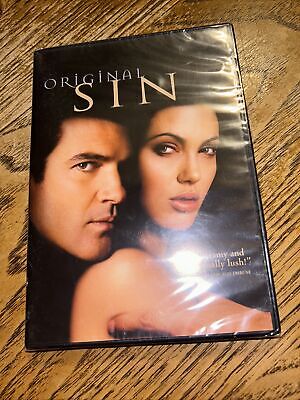This is a detailed photograph of a DVD cover for the movie "Original Sin," featuring Hollywood stars Antonio Banderas and Angelina Jolie. The cover displays a black background with the title "Original Sin" written in gold across the top. The picture on the cover depicts Banderas and Jolie from the shoulders up; Jolie appears to be naked with bare shoulders and arms, while Banderas stands behind her in a shadowed area. Both have dark hair and dark eyes, and they are looking sideways, slightly towards the viewer. The DVD cover lies on a light to medium stained wooden surface with visible wood grain and black lines. A camera flash creates a reflection on the bottom right corner, partially obscuring additional text.